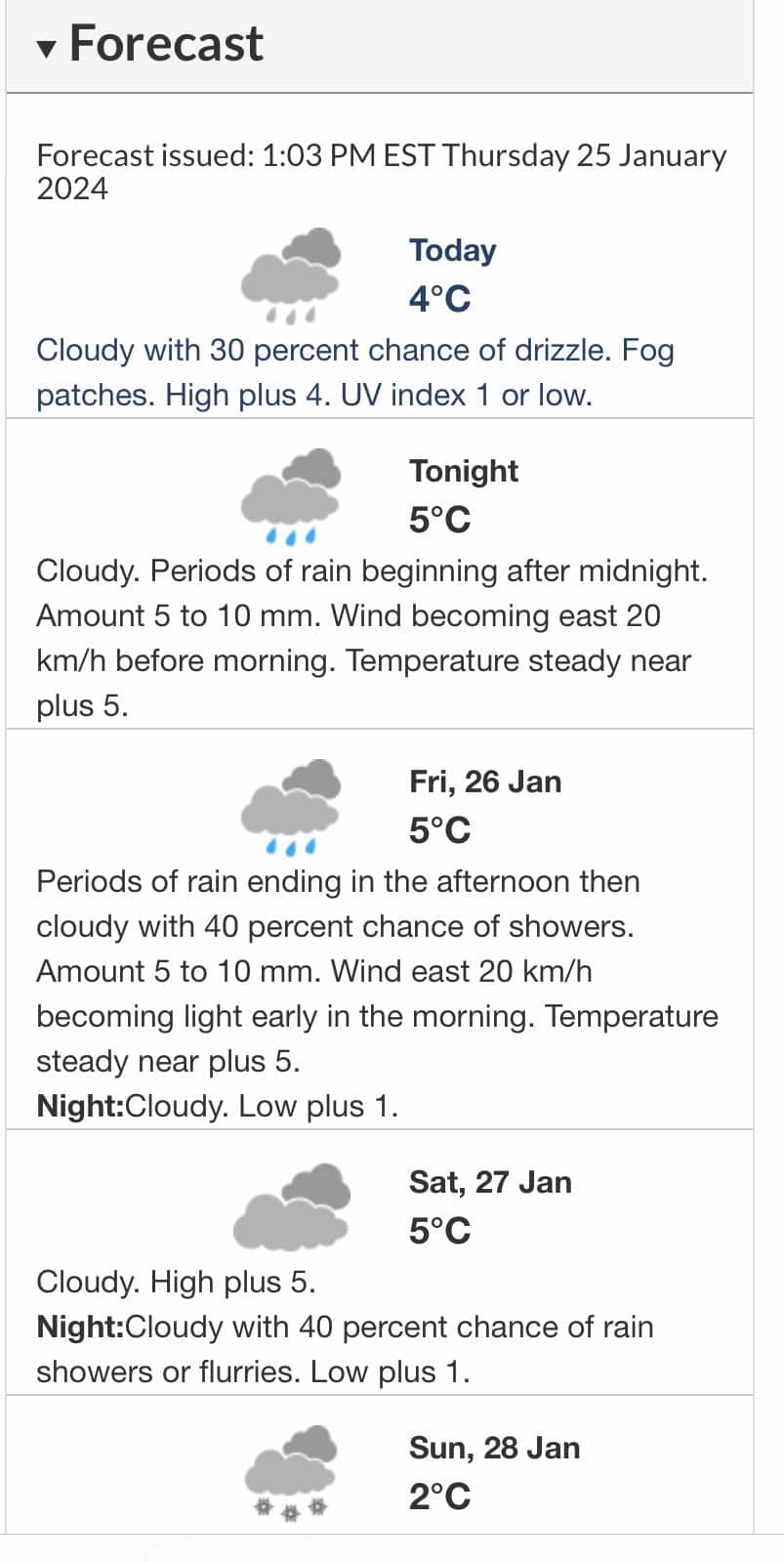In the provided image, we see a screenshot of a weather forecasting application designed for a mobile device. At the top of the interface, the word "Forecast" is prominently displayed alongside a down arrow button, indicating a dropdown menu for additional options or settings. Beneath this header, various weather notifications and updates are listed.

The forecast was issued at 1:03 PM Eastern Standard Time on Thursday, January 25, 2024. A graphic illustrating gray clouds with raindrops accompanies the text for a visual representation of the weather conditions.

The detailed weather information reads as follows:
- **Today:** The temperature is 4 degrees Celsius with an overall cloudy sky and a 30% chance of drizzle. Fog patches are also mentioned. The high is expected to be plus 4 degrees with a UV index of 1, categorized as low.
- **Tonight:** The temperature is projected to be 5 degrees Celsius with cloudy conditions and periods of rain beginning after midnight. The expected rainfall amounts to around 5 to 10 millimeters. Winds are anticipated to shift, becoming eastward at 20 kilometers per hour before morning. The temperature is expected to remain steady near plus 5 degrees Celsius.
- **Friday, January 26th:** The temperature will be 5 degrees Celsius with periods of rain continuing into the afternoon before turning to a cloudy sky with a 40% chance of showers. The total rainfall is estimated to be between 5 to 10 millimeters. A visual icon depicting clouds and yellow raindrops accompanies this forecast.
- **Saturday, January 27th:** The forecast extends to another day, with the temperature expected to remain at 5 degrees Celsius.

Each forecast period is accompanied by appropriate weather icons for visual clarity, aiding users in quickly grasping the expected conditions.